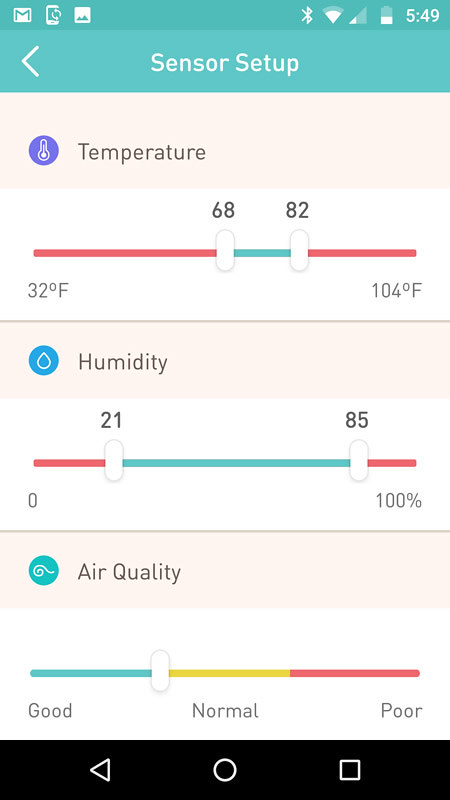This is an image of a sensor setup interface displaying various environmental parameters. The interface includes controls for temperature, humidity, and air quality. The temperature settings range from a minimum of 68°F to a maximum of 82°F. For humidity, the minimum is set at 21% and the maximum at 85%. Additionally, there is a slider to adjust air quality, which is currently positioned between "Good" and "Normal." The UI provides a comprehensive overview and control of these environmental factors.